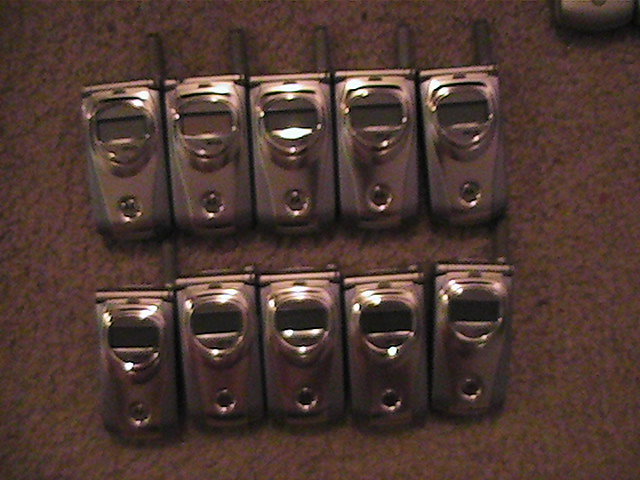The photograph is an overhead shot of a dark, grainy setting featuring ten flip phones arranged on a dingy, dark gray carpet. The phones are organized into two rows of five. The top row consists entirely of identical silver flip phones with small black antennas on the top right and a rectangular display window in the middle. The bottom row has the same silver flip phones, but only the ones on the bottom left and bottom right have antennas; the three in the middle are missing their antennas. Additionally, in the upper right corner of the image, there is a partial view of an extra flip phone, silver like the others, contributing to the image's scattered, old-school tech aesthetic.